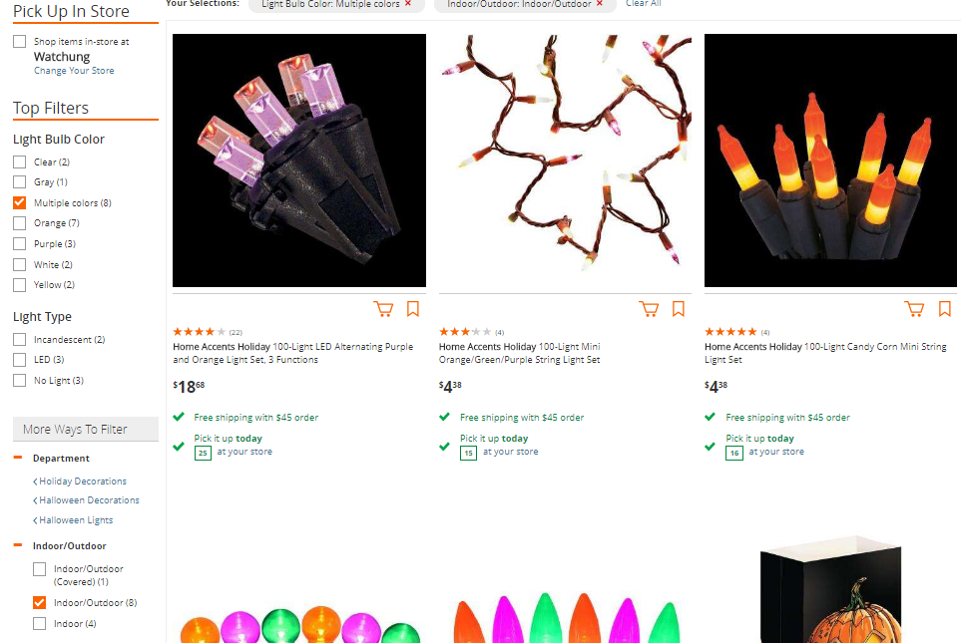The screenshot showcases a webpage for a store, specifically highlighting various holiday light sets available for purchase. 

- **First Option:**
  - **Product:** Home Accent Holiday 100-Light LED Alternating Purple and Orange Light Set
  - **Features:** Three lighting functions
  - **Price:** $18.68
  - **Shipping Information:** Free shipping on orders over $45.00 or available for same-day pickup at the store
  - **Reviews:** Rated 4 stars

- **Second Option:**
  - **Product:** Home Accent Holiday 100-Light Mini Orange Green Purple String Light Set
  - **Price:** $4.38
  - **Shipping Information:** Free shipping on orders over $45.00 or available for same-day pickup at the store
  - **Reviews:** Rated 3 stars

- **Third Option:**
  - **Product:** Home Accent Holiday 100-Light Candy Corn Mini String Light Set
  - **Price:** $4.38
  - **Shipping Information:** Free shipping on orders over $45.00 or available for same-day pickup at the store
  - **Reviews:** Rated 5 stars